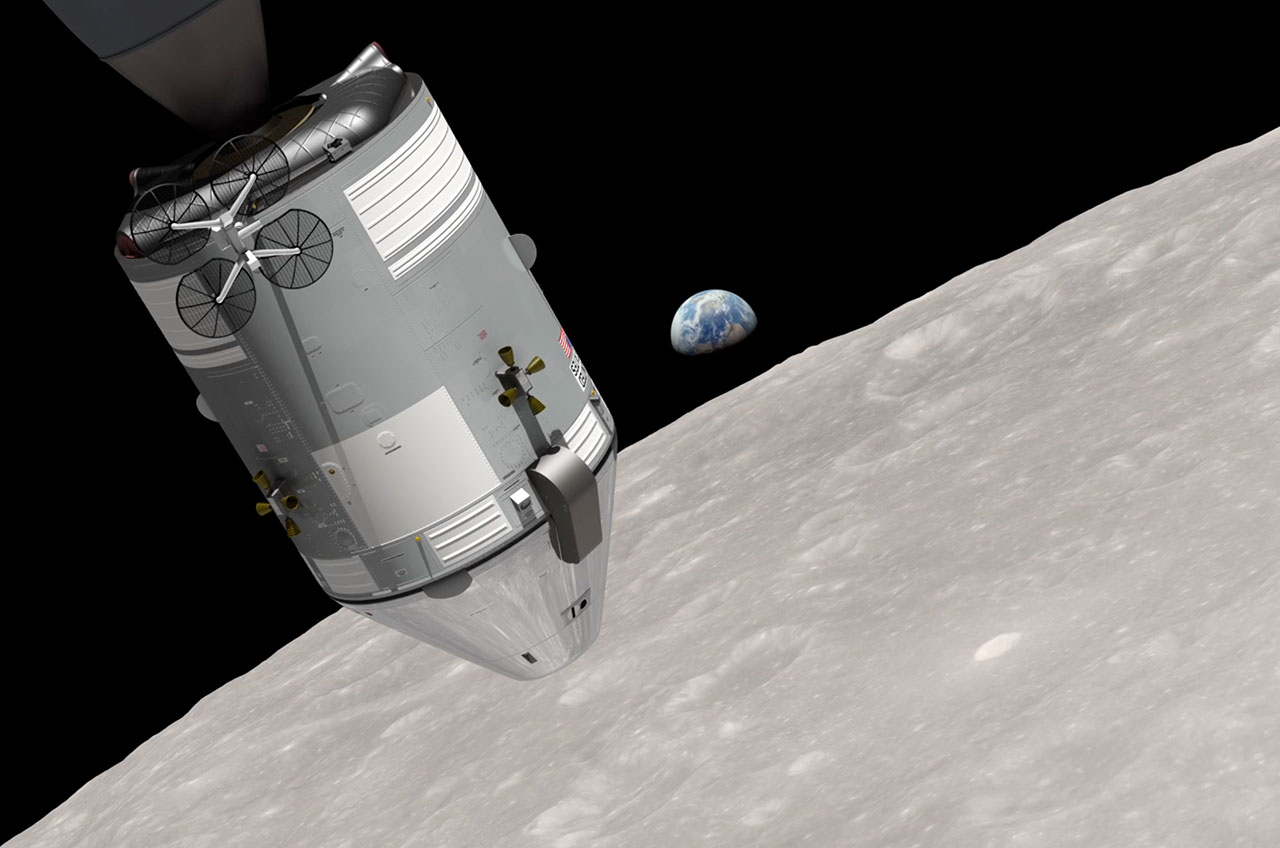The digital image depicts a scene in outer space featuring a space capsule floating above the moon. The capsule is predominantly gray with some white patches, adorned with cross-like golden elements. It has a cylindrical body ending in a pointed, metallic chrome cone. The capsule is positioned towards the left side of the image, with the cone oriented slightly downward to the right. 

In the foreground, the moon's silvery gray surface stretches from the bottom left corner to the upper right side, detailed with numerous craters and some white spots. In the background, the Earth is visible, about three-quarters of it showing as a vibrant blue and white globe, partially shrouded in darkness with visible clouds. The dark, black void of space forms the backdrop, accentuating the celestial elements.